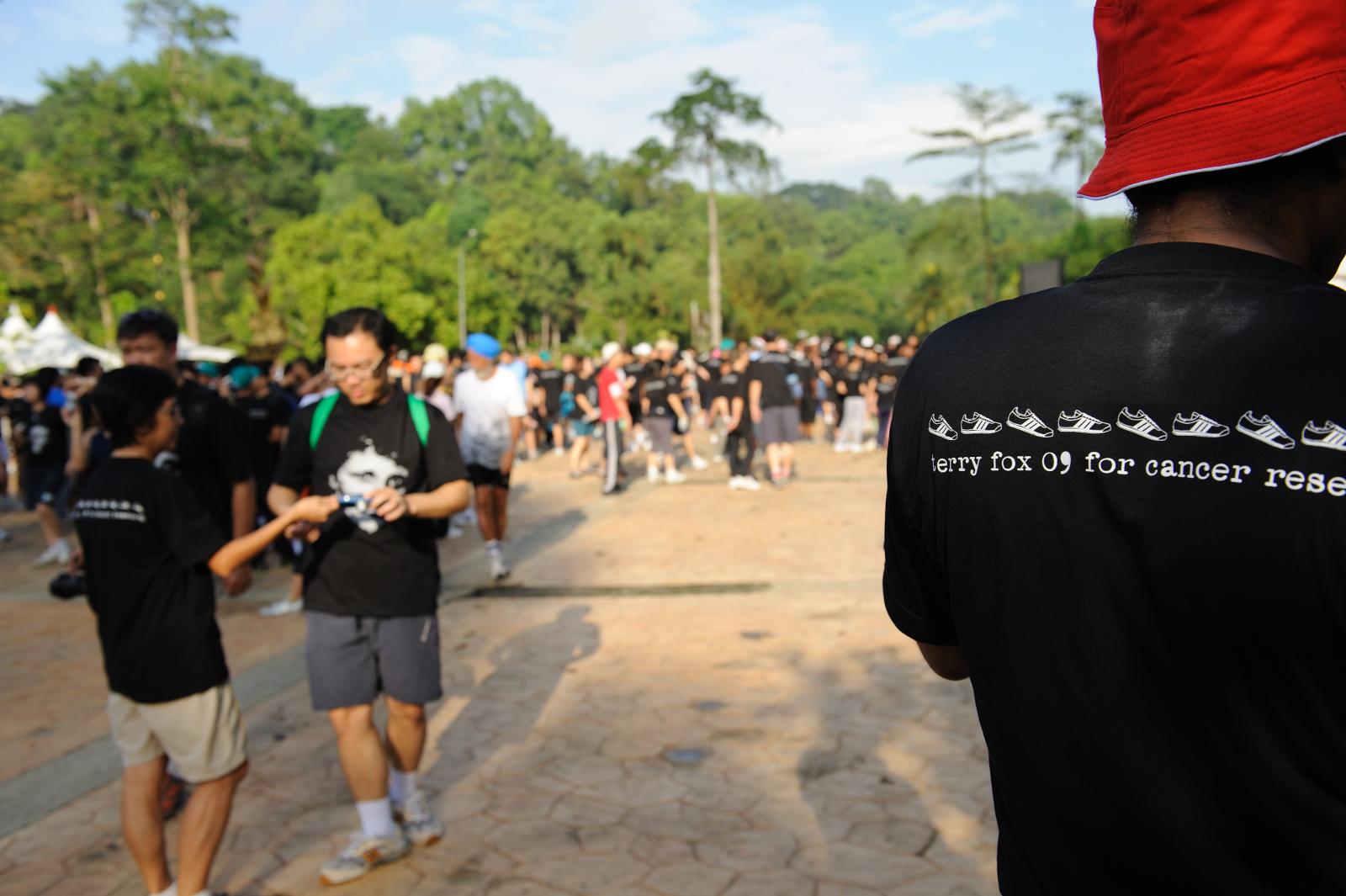The photograph captures a lively gathering of people in a stone courtyard, enveloped by dense trees under a partly cloudy sky. Many of the attendees, including a man on the right in a red cap, are wearing the same black t-shirts that read "Jerry Fox 09 for Cancer Research" with an image of Adidas soccer shoes adorned with the brand's three stripes above the text. This suggests that it's a cancer research event, likely named in honor of Jerry Fox. Towards the left, there are some tents that hint at merchant stalls or informational booths. The various people, engaged in walking and conversation, add a dynamic quality to the scene, indicating that it's likely midday during some sort of run for cancer research. The predominant colors in the image are black, red, blue, green, and gray, contributing to the vibrant atmosphere of the event.